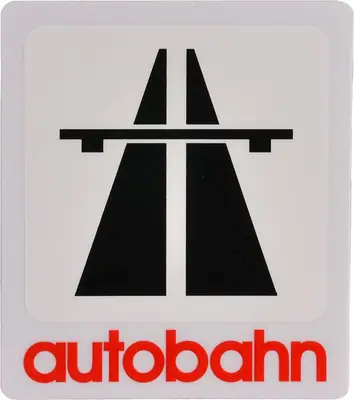The image is slightly taller than it is wide and features a light brown border with rounded corners. The background within this border is a grayish off-white color. At the bottom of the image, in bright red lowercase letters, is the word "Autobahn," which spans the entire width of the image. Above the text, centered within a smaller, slightly different colored gray box, there is a symbol. This symbol comprises two black vertical lines that are intersected midway by a horizontal line, resembling a bridge crossing over a road. Additionally, the symbol includes two right triangles positioned next to each other, flanking the vertical lines. This detailed imagery suggests that the sign serves as a recognizable logo or road sign indicating the Autobahn.